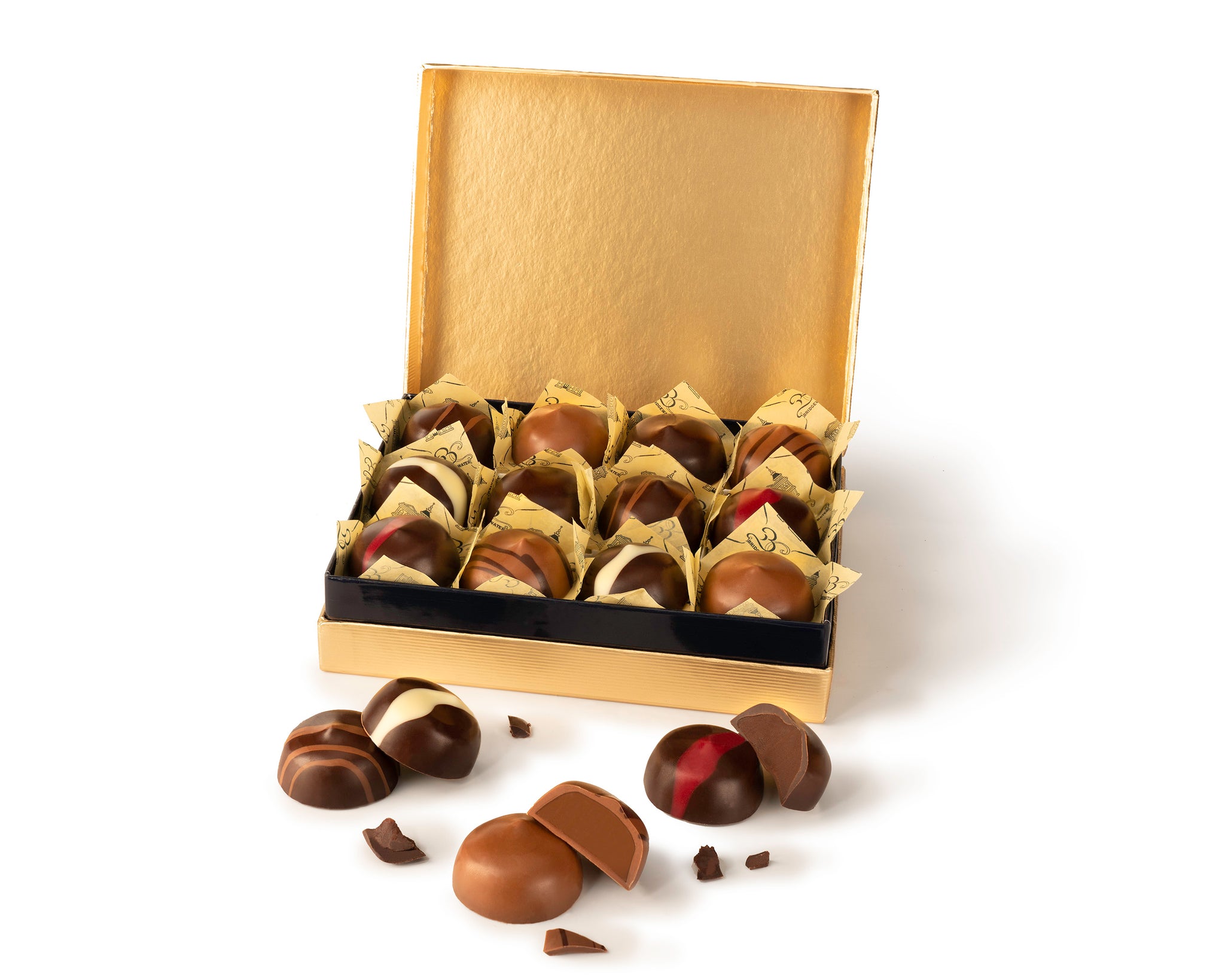The image showcases a meticulously arranged gift set of chocolates against a pristine white background. At the center, an open black and tan gift box is slightly tilted to the right, unveiling an inner golden and brown container that securely holds twelve individually wrapped chocolates. These chocolates are neatly organized in a four-by-three grid, each enclosed in light yellow tissue paper. Positioned above the bottom part of the box is the detached top lid. Below the box, on the white surface, lie several chocolates, some intact and some partially bitten, with a few broken pieces nearby, offering a glimpse of their varied fillings. The overall presentation emphasizes the elegance and appeal of the chocolate gift set.